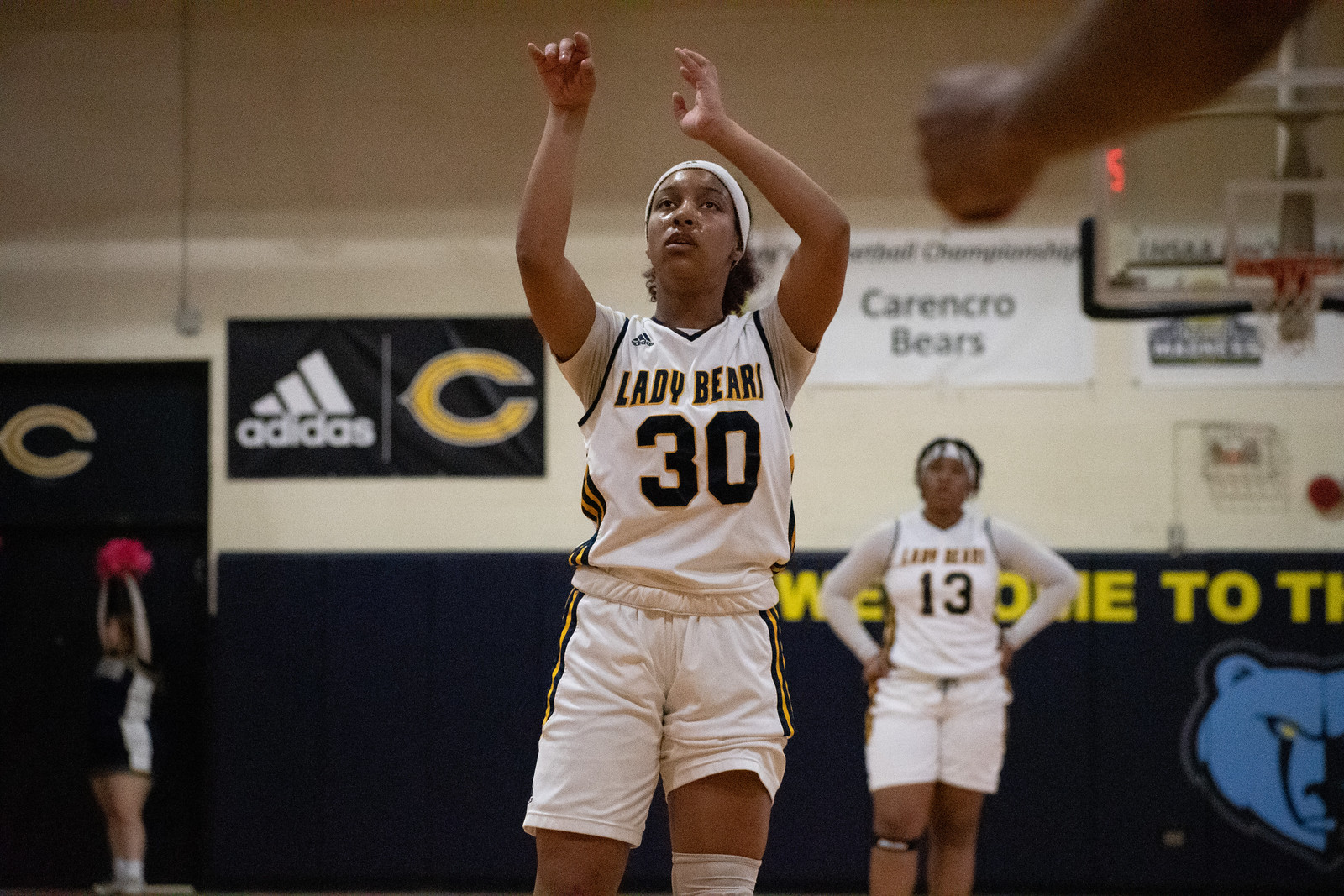In the gymnasium, two African American female basketball players in white uniforms numbered 30 and 13 stand facing the camera. Their jerseys read "Lady Bears" with black numbers outlined in yellow, and feature the Adidas logo. The player with the number 30 is closest to the camera, wearing a white headband and an ace bandage on her knee, while the number 13 player stands further back with her hands on her hips. Both uniforms have red and black piping on the sides. 

The gym's tan wall is adorned with several banners, including one that displays the Adidas logo alongside the letter 'C', and another that reads "Karen Crow Bears." Below these, a lower blue backdrop features the message "Welcome to The" along with an animated image of a bear's head. On the left side of the image, a cheerleader wearing a black uniform with white stripes holds a red pom-pom overhead. A basketball hoop and scoreboard are also partially visible, emphasizing the indoor sports setting.